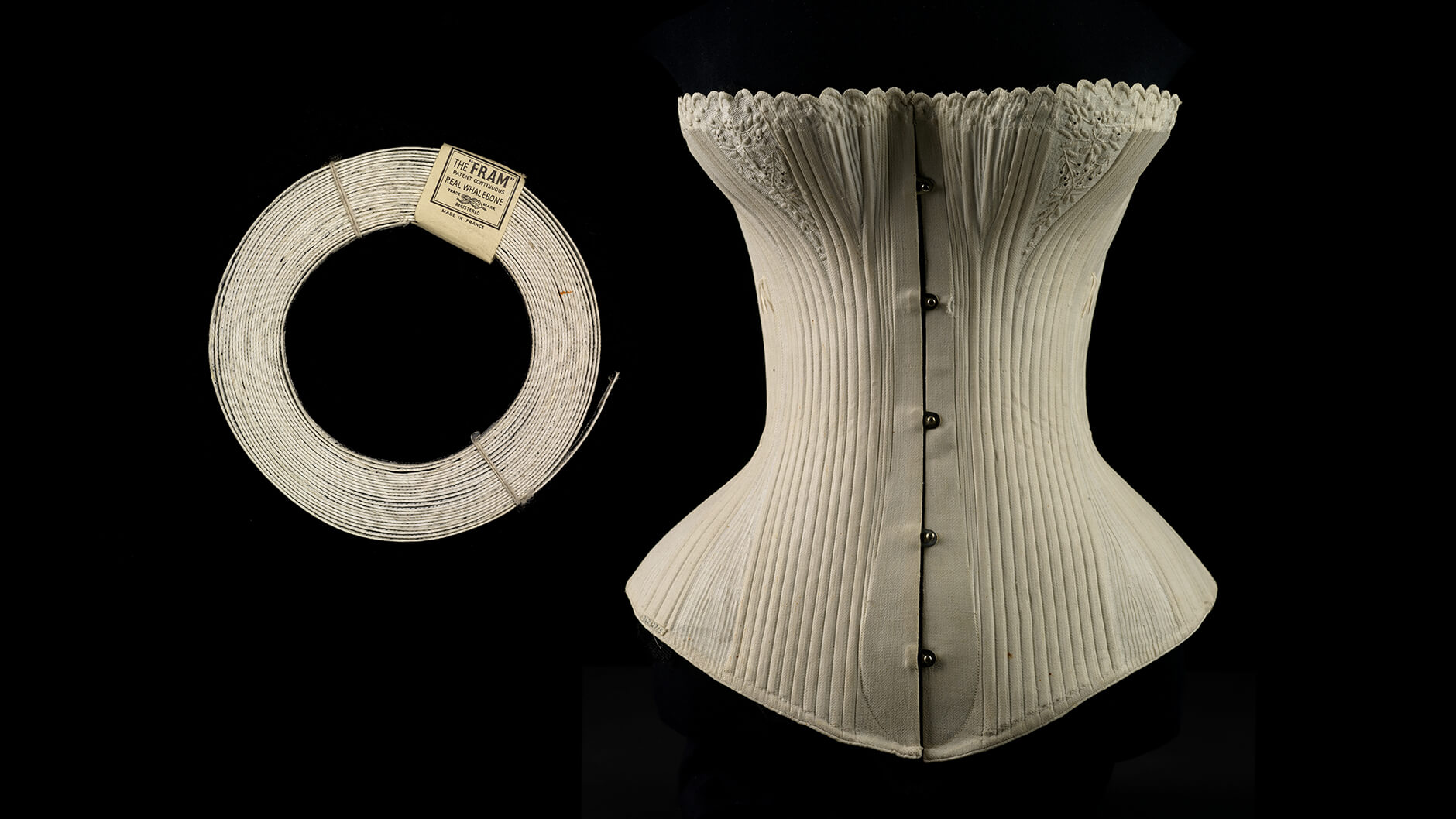This detailed image showcases a vintage beige corset contrasted against a black background. The corset, positioned on the right, displays an aged white hue and is designed with an hourglass shape: a fitted waist, an expansive bust area, and a wide lower section. Five button hooks run centrally down the piece, adding to its intricate design. The upper portion near the bust features a fluted, frilly texture that enhances its ornate appearance. On the left side of the image, there is a bundle of white string or perhaps lace, possibly folded rope, tied in two spots for neatness. A beige tag attached to this string reads "the frame," followed by "real whalebone" in black text, hinting at the corset's authentic materials and possibly indicating it is made in France. This piece seems to be DIY-friendly, offering the materials and instructions for personal assembly.